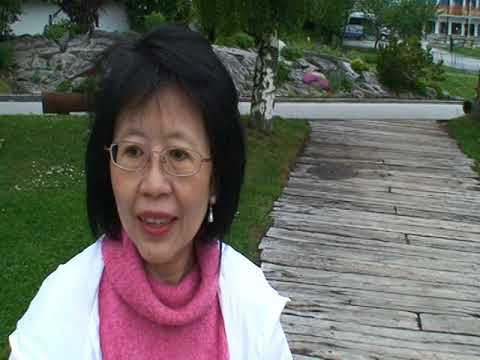The image depicts an overcast outdoor scene featuring an older Asian woman with dark shoulder-length hair and glasses standing slightly to the left of the frame. She wears a pink turtleneck sweater with a saggy neck and a white jacket over it. Her accessories include thin wire-frame glasses, pink lipstick, and small pearl earrings. In the foreground, a grassy area is bisected by a wooden plank walkway. Behind her, at the end of the walkway, there is a paved street bordered by a small, modeled tree with a white and green trunk and thin leaves. Across the street, a landscaped hill features gray stones, bushes, and flowers. In the background, on the far right, stands a tall two-story white building with columns.